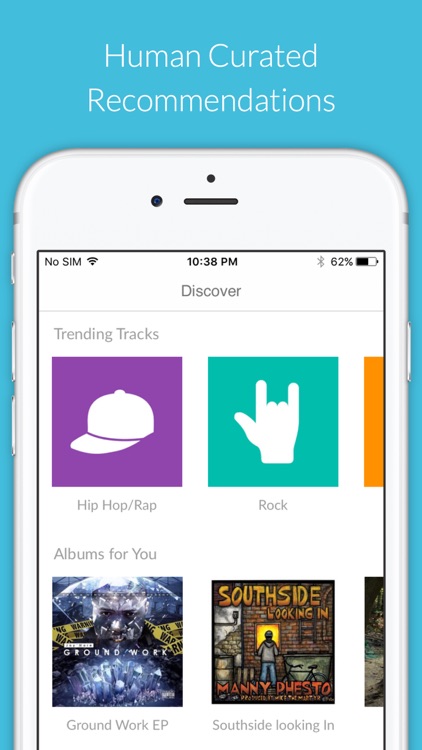A detailed and clear caption for the image could be:

---

A close-up image of a white smartphone is centered against a light blue background. The top of the smartphone screen displays white text that reads "Human Curated Recommendations." Directly below this text, the phone shows various status icons and information, including "No SIM," a Wi-Fi signal icon, the time "10:38 PM," a Bluetooth icon, and "62% battery." Beneath these details, the screen displays the word "Discover" followed by a light gray horizontal line. Below the line, the heading "Trending Tracks" is prominently featured. Under this heading, there is a purple rectangle with a white baseball cap icon accompanied by the text "Hip Hop / Rap." Further down, the screen showcases an album titled "Groundwork EP," depicted as a white, yellow, and blue image that is too blurry to make out clearly. To the right of this album, the text "Southside Looking In" appears, credited to an artist named "Manny Doe" (or something similar), with the album title "Southside Looking In" reiterated below.